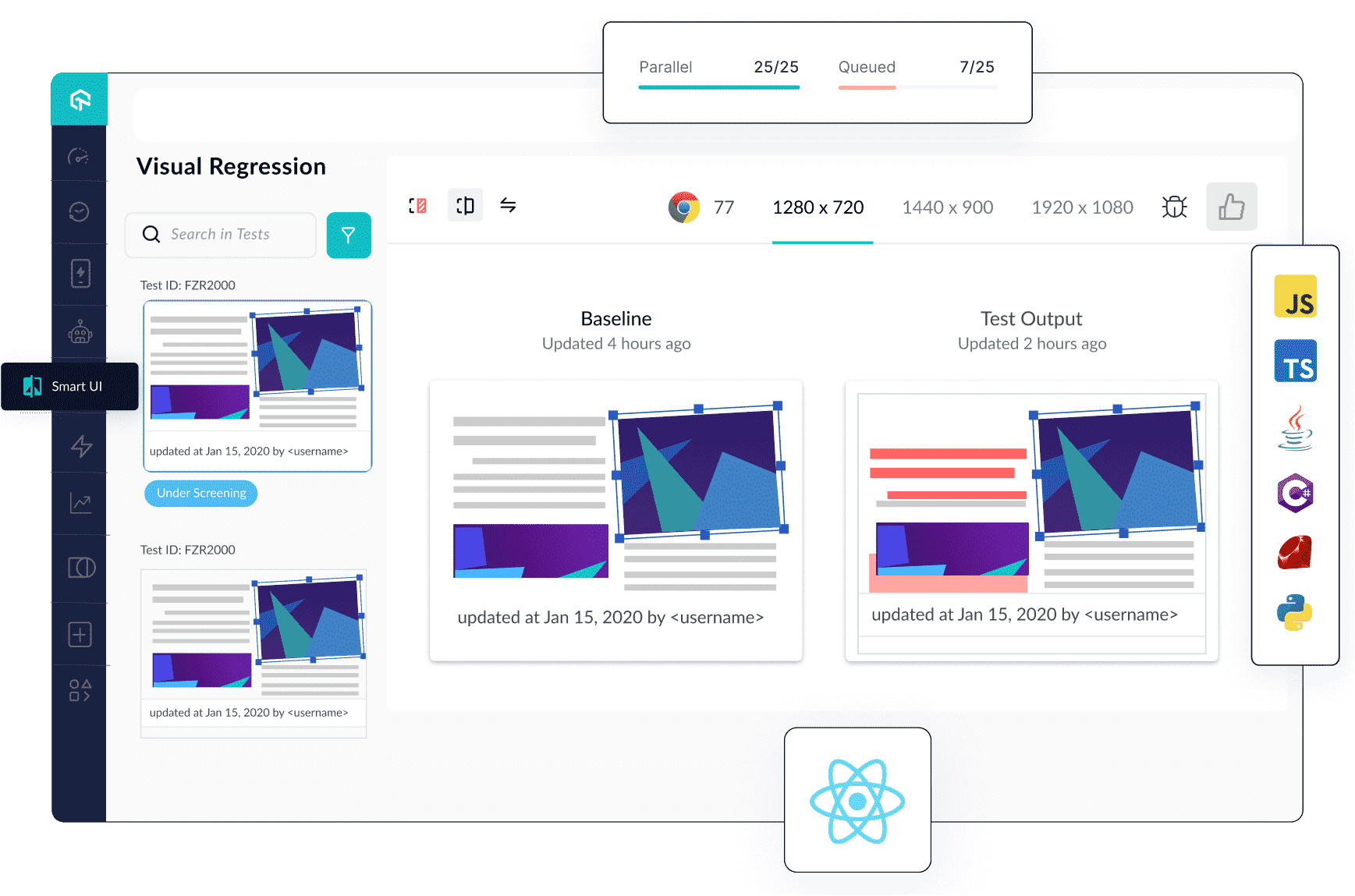The image depicts an open application or website window on a computer screen, specifically showcasing a user interface focused on "Visual Regression." 

On the left-hand side, there's a sleek, dark gray vertical sidebar extending from the top to the bottom of the window. This sidebar features 11 distinct icons arranged vertically, though their specific functions are not immediately recognizable. The active tab within this interface is titled "Visual Regression," with the label rendered in black text, indicating its selection. Directly below this, there is a "Search in text" field accompanied by a blue search link.

At the top of the screen, a pop-up menu displays two statuses: "Parallel 25/25" and "Queued 7/25." Each status is elucidated with progress bars, where the 'Parallel' progress bar is fully complete at 25 out of 25, while the 'Queued' bar indicates progress with 7 out of 25 completed.

Below these status indicators, a series of links appear, likely offering various adjustments or settings related to the content or process being worked on. The content of the workspace includes a specific project or item categorized as "Baseline," which was updated four hours ago. Another item in the workspace is labeled "Text Output," which was updated two hours ago.